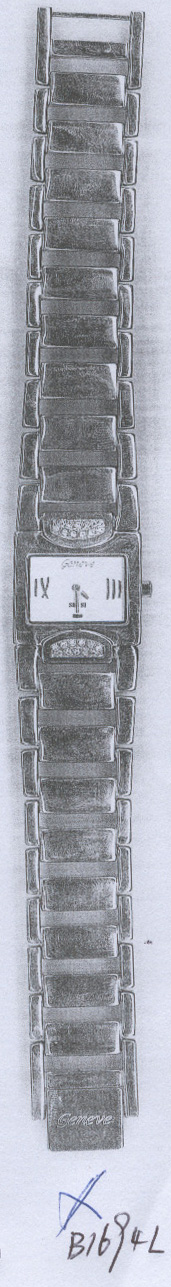This piece appears to be a photograph of a grayscale drawing on white paper, featuring a detailed, photorealistic depiction of a slender, chain-link watch band. The band resembles a silver chain with intricately shaded links, rendered in shades of gray and dark gray. At the center of the band sits a small, white, square watch face. The watch face displays the time as 4:30, with visible minute and hour hands, and shows Roman numerals on the left and right edges of the square. The watch face also has inscriptions in a different language and a visible pin on the right side. Beneath the watch band, there is a blue signature followed by the characters "B-I-B-E-G-4-L" written in black. The artwork also exhibits a pin along with horizontal lines and squares, suggesting detailed craftsmanship in the drawing.